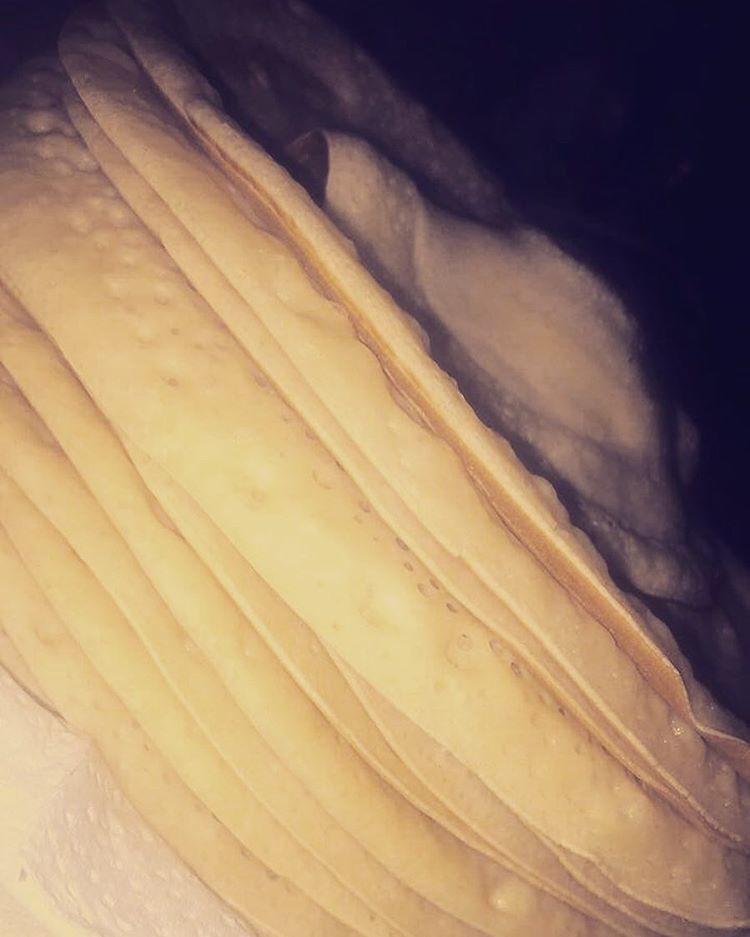The image is an extreme close-up color photograph of a stack of pale yellow crepes, taken at an angle that makes the layers appear diagonal and somewhat harder to identify at first glance. The stack consists of approximately 10 to 11 crepes. The background is mostly dark, with a black upper right corner providing little context of the surrounding environment. The top crepe in the stack seems to be either being lifted off or placed onto the stack, creating a slight separation from the rest. In the bottom left corner, there is a white object that could be either another crepe, a plate, or a paper towel, partially visible and adding to the ambiguous tactile elements of the composition.